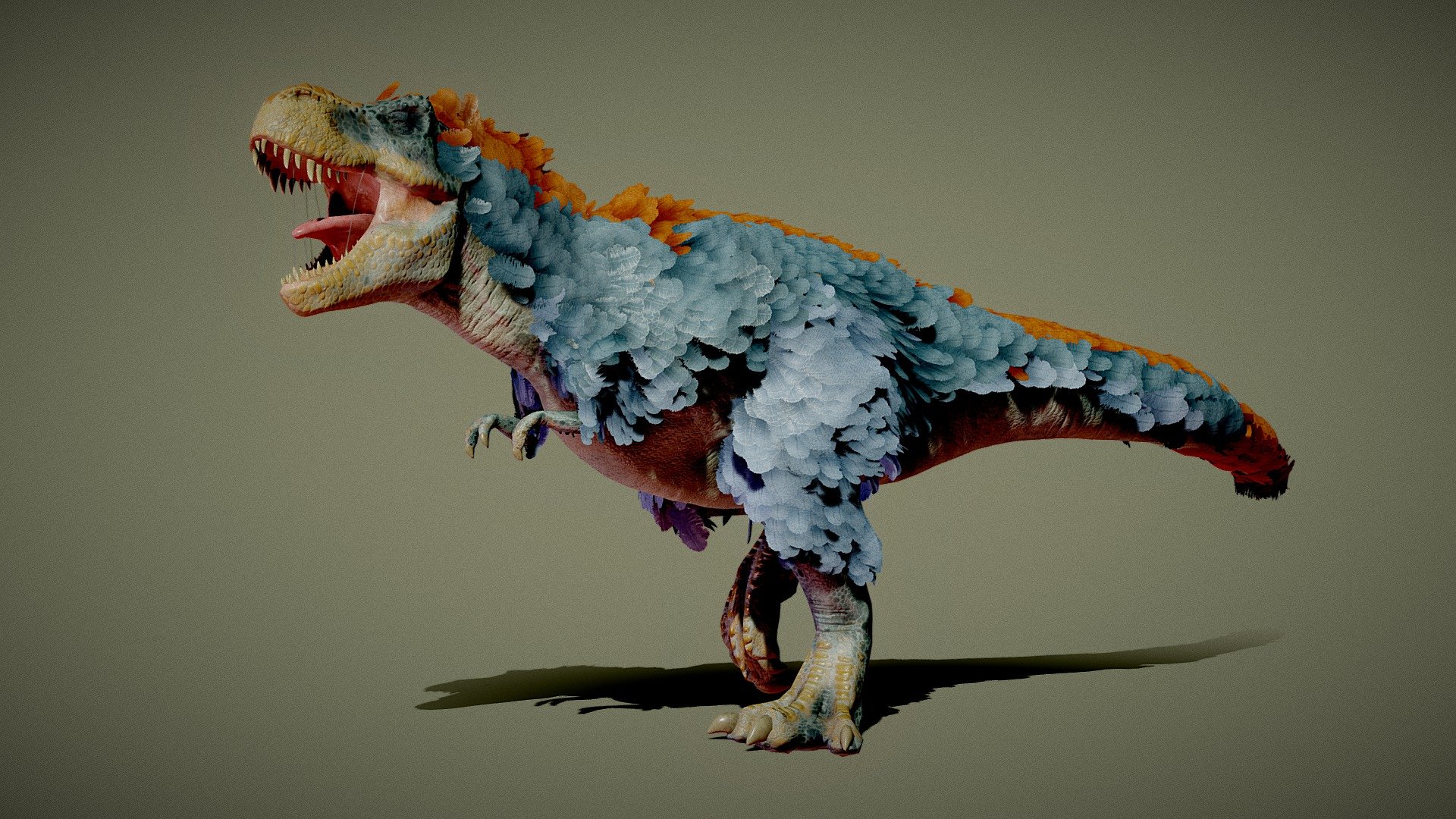The image showcases an intricately detailed depiction of a Tyrannosaurus rex, set against a dark gray or olive-toned background. The creature's mouth is wide open in a roaring stance, revealing sharp teeth and a thrust-out tongue, giving a sense of ferocity as it faces left. Rendered with meticulous attention, the T-Rex is adorned with an unusual and fascinating coat of feathers. These feathers are primarily a light blue or turquoise color, covering the body but leaving the feet, hands, head, and throat bare. Along its back and tapering down to the tail, there is a striking display of orange feathers, contrasting vividly with the bare red belly. Small, characteristic arms extend out front, adding to the lifelike posture. The image appears to be highly realistic, possibly a photograph of a detailed model or an exceptionally well-rendered piece of digital art, emphasized by the shadow cast on the ground below. This depiction aligns with modern scientific theories suggesting that some dinosaurs, including the T-Rex, might have been covered with feathers.